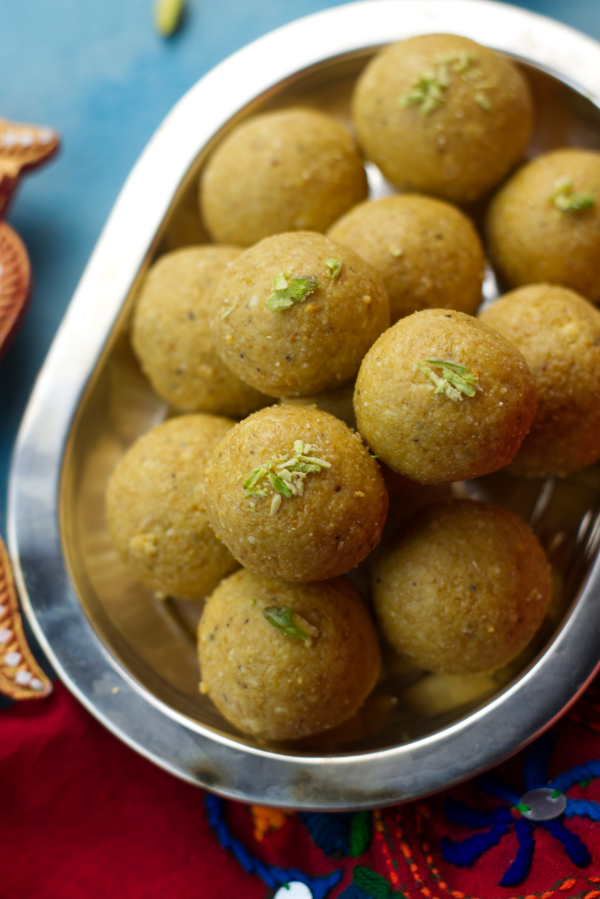This photograph captures an aerial view of an oval-shaped silver vessel, diagonally positioned, containing several round, deep-fried food items akin to risotto balls or arancini. These golden-brown spheres, possibly savory cultural treats, are modestly garnished with green herbs. The vessel rests on a red felt placemat adorned with blue floral patterns. To the side, a blue background features a partially visible orange vase. The setting suggests a vibrant and inviting dining experience, rich in color and texture.